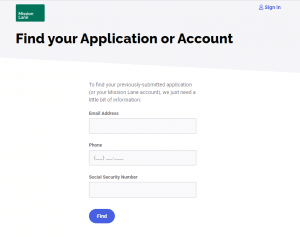The image depicts a user interface for account access on a light blue header against a white background. At the top of the header, there is a profile symbol accompanied by the text "Sign In" in blue. Below, a green rectangular button prominently features two words in white text. Further down, the interface displays a section for entering user information. There are input fields labeled "Email Address" and "Phone," with the phone number formatted as three parentheses-enclosed digits followed by three additional digits, a dash, and finally four more digits. Another input field is labeled "Social Security Number." At the bottom of the interface, there is a blue oval button containing the word "Find" in white text.